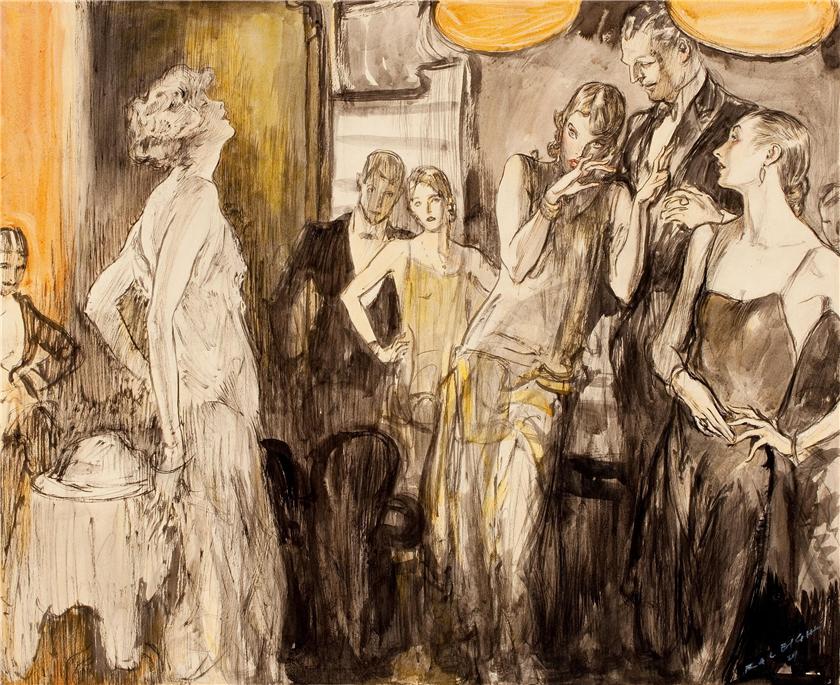The image is a detailed, old-fashioned graphic, hand-drawn or painted, likely depicting a scene from the 1920s or 1940s. The ambiance suggests a fancy ball or formal gathering. Men are dressed in elegant suits and ties, while women wear long, form-fitting evening gowns, with their hair styled in vintage updos. The color palette includes shades of black, white, yellow, orange, tan, and brown. The setting features decorated tables, some with silver food covers, and chairs draped in tablecloths. The ceiling is adorned with hanging balloons, adding to the festive atmosphere.